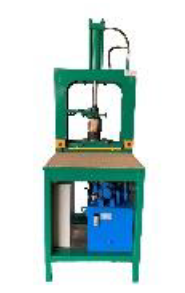The image depicts a piece of workshop machinery with a predominantly dark green, upright frame that resembles a large chair. This machine seems to be designed for pressing objects, though its exact purpose is unclear. The structure includes a main work area where items can be placed, characterized by a light brown tabletop. Extending through the middle of the setup is a metal component that appears to be part of a drill or pump mechanism, incorporating copper or metal elements with green tubing attached. 

Near the bottom of the machine, there is a shelf housing a few components—a blue motor with black hoses connected to it, and a large white semi-cylinder object. The machine also features a square-like frame in the background, and there is a case that can be opened to access the internal parts for maintenance. Various pipes and hoses run throughout the system, contributing to its complex appearance.